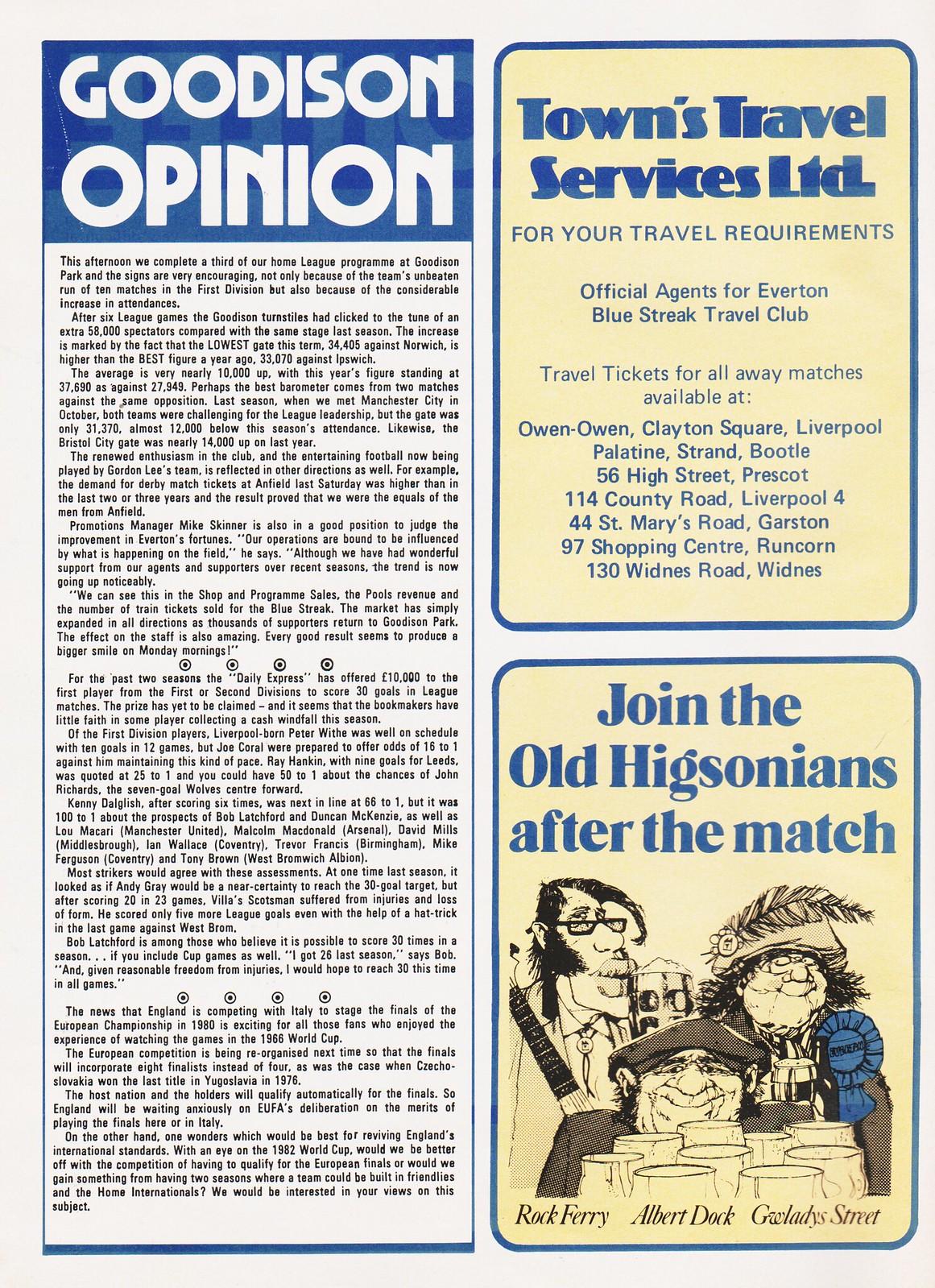The image depicts a page from a pamphlet or magazine, featuring a prominent opinion piece titled "Goodison Opinion" on the left-hand side against a white background. The opinion piece is structured in several paragraphs and enclosed within a blue border. On the right-hand side of the page, there are two vertical advertisements. The top ad, with an ivory-colored background and blue text, promotes "Towns Travel Services, LTD" for travel requirements, specifying that they are official agents for Everton Blue Streak Travel Club and providing details about ticket availability. Below it, another ad with a blue border and blue text invites readers to "Join the Old Higsonians After the Match," accompanied by a sketch of three people in a bar, labeled as Rock, Ferry, Albert, and possibly Gladys. The overall style suggests a structured layout typical of a football-related pamphlet, blending editorial content with thematic advertisements.